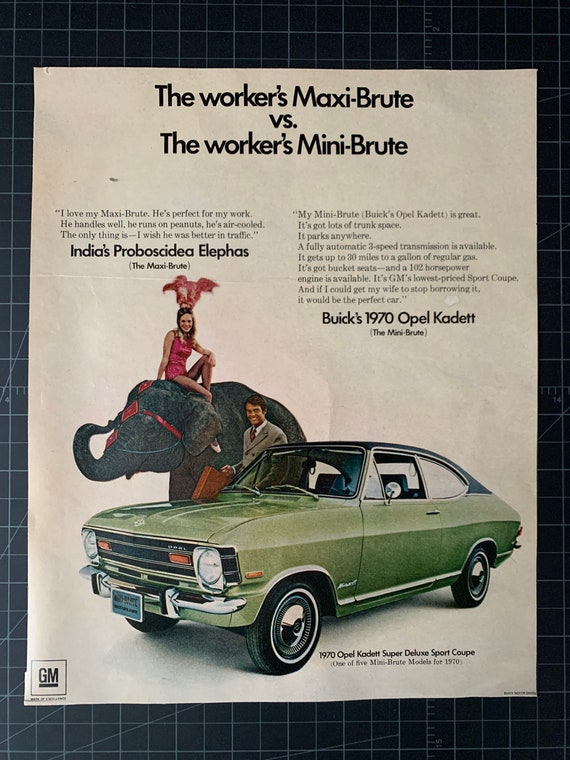**Vintage Advertisement for Vehicles: The Worker's Maxi-Brew vs. The Worker's Mini-Brew**

At the top of the advertisement, the headline reads: *"The Worker's Maxi-Brew vs. The Worker's Mini-Brew"* in bold black font. Below this, a testimonial for the Maxi-Brew states:

*"I love my Maxi-Brew. He's perfect for my work. He handles well, runs on peanuts, and is air-cooled. The only thing is, I wish he was better in traffic."*

Accompanying this quote is an illustration of an imposing elephant with a woman dressed in red comfortably seated atop it, capturing the essence of strength and capability of the Maxi-Brew. Underneath this image, the tagline proudly declares: *"India's Propitiated Alpha, the Maxi-Brew."*

To the right, another quote extols the virtues of the Mini-Brew:

*"My Mini-Brew, Buick's Opie Cadet, is great. It's got a lot of trunk space, parks anywhere, and a fully automatic three-speed transmission is available. It gets up to 30 miles per gallon of regular gas, has bucket seats, and a 102-horsepower engine is available. It's GM's lowest-priced sports coupe. If I could get my wife to stop borrowing it, it would be the perfect car."*

This quote is accompanied by an illustration of a sleek, green coupe vehicle, epitomizing the modern, practical, and economical features of the Opie Cadet.

At the bottom left corner of the advertisement, the recognizable GM logo is prominently displayed, underscoring the brand's legacy and reliability.

**Note:** All objects and text appear to be upright and meticulously aligned, showcasing the advertisement's structured and well-thought-out design.